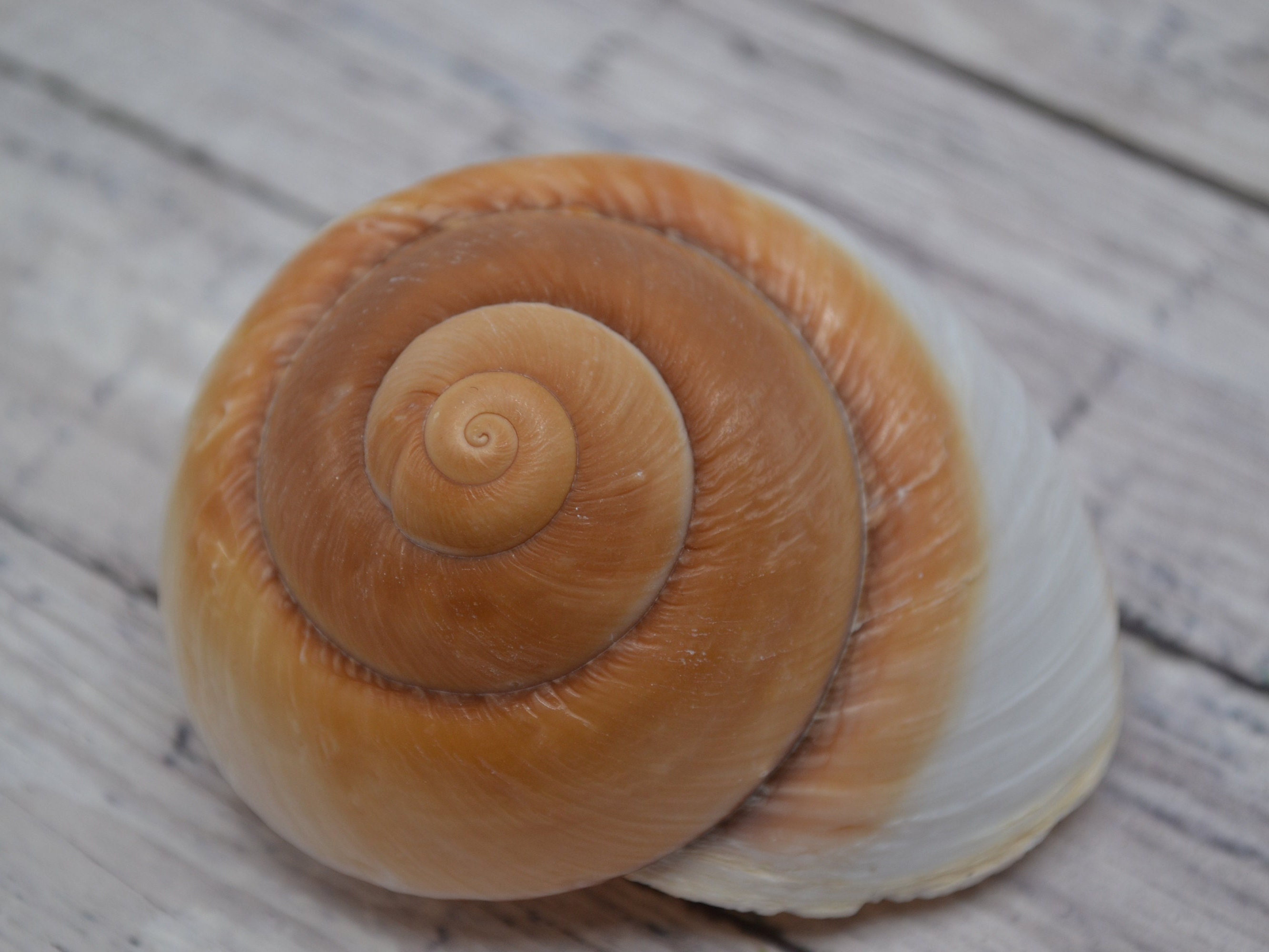The image is a close-up, color photograph of a seashell, focusing on intricate details. The image, rectangular in shape and about six inches wide by four inches high, showcases the shell as the central element on a light-colored wooden surface with diagonal slats, likely a porch or deck, in shades of light gray and bits of light brown. The seashell is spiral-shaped, measuring approximately three inches high and four to five inches wide. It features a smooth texture with striations, starting with a white-toned outer ridge that transitions to medium brown and light beige colors. The spiral begins at the bottom right, curling outward and upward to the left, then tightening into the finest, tiniest shape in the center with darker brown along the spiral edges and a lighter brown re-emerging in the middle.